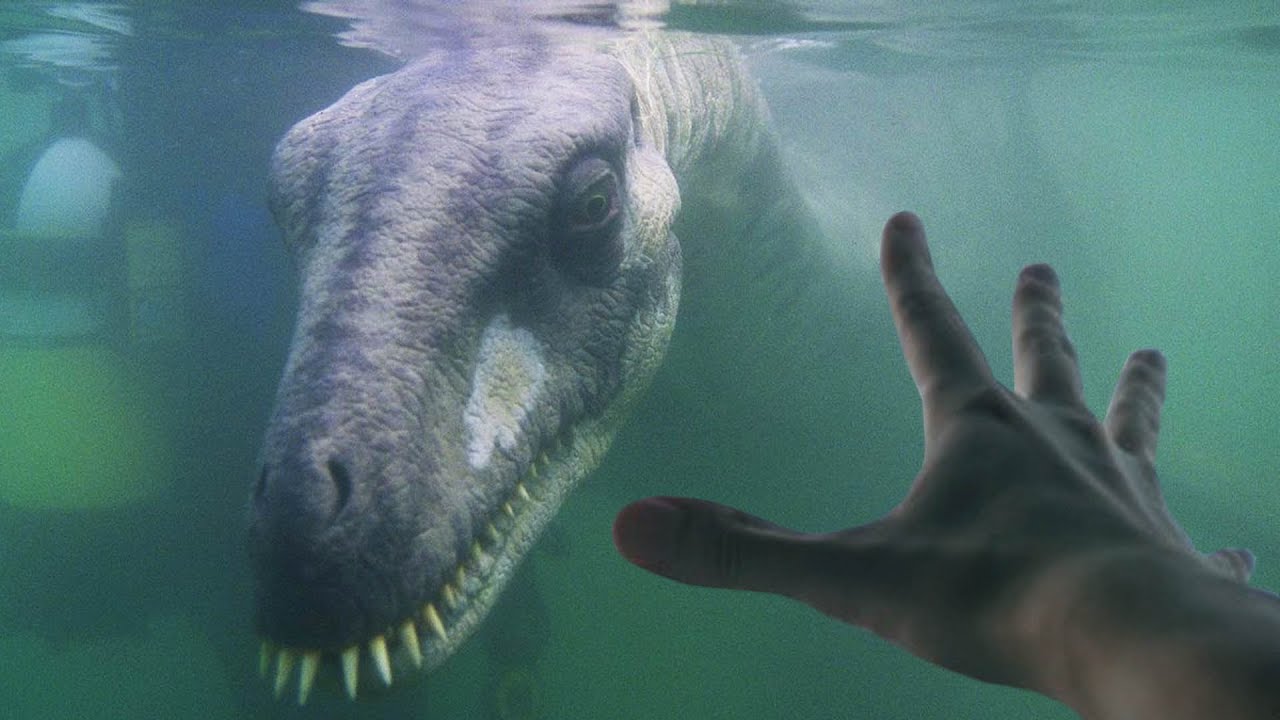The image appears to be an AI-generated scene featuring a close-up of a dinosaur-like creature in an aquarium tank filled with murky, greenish-blue water. The dinosaur's head and part of its neck are visible, with its body disappearing into the cloudy water. The skin of the dinosaur is scaly and textured, exhibiting a mottled pattern of darker and lighter browns, though some descriptions suggest a grayish or bluish tint with lighter spots around the neck. Prominently, there is a distinctive white splotch on the left side of its face, with hints of blue and yellow near its eye. The creature's mouth is closed but filled with numerous sharp, spiky white teeth that protrude visibly. A human hand, with thin fingers fully outstretched, is pressed against the glass in the bottom right of the frame, reaching toward the dinosaur as if attempting to touch it. The hand and the dinosaur create a striking juxtaposition, emphasizing the eerie, surreal quality of the scene.